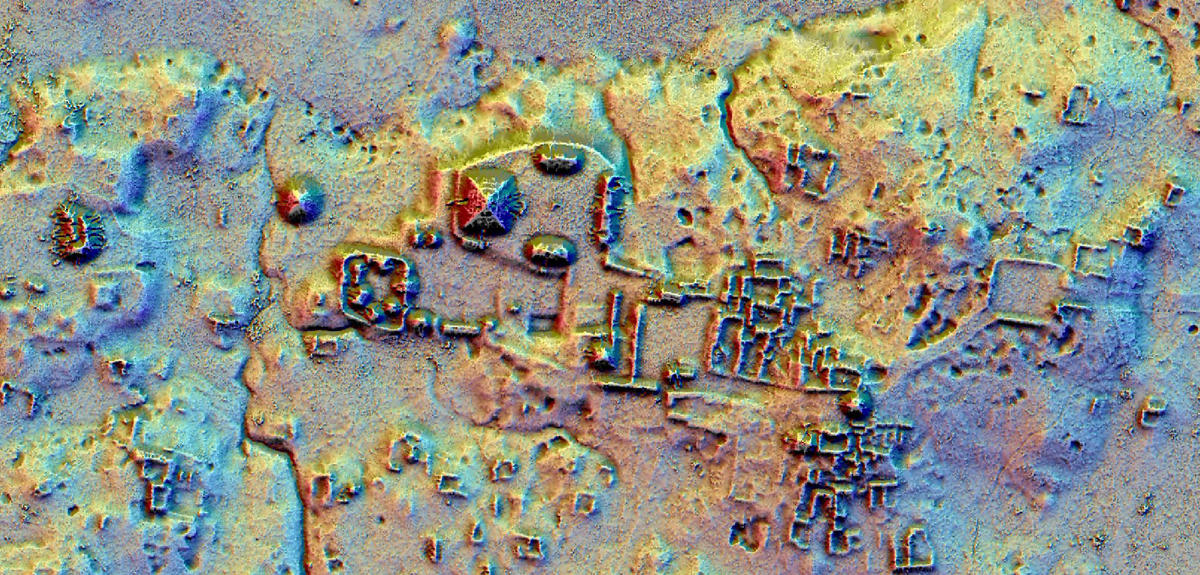This image is a detailed ground-penetrating radar result, displaying various elevations within an ancient archaeological site. The radar image, composed of vivid hues including blue, violet, red, yellow, and orange, reveals the intricate layout of what appears to be a historic village or city. At its center is a prominent square or rectangular structure, indicative of a primary building or pyramid. Surrounding this central feature are numerous smaller structures, including triangular-shaped elements suggesting walls and rooms. The outer regions of the image transition to a grayish-blue color, while the center bursts with red and yellow tones. This heat map visualization highlights the complex spatial arrangement of buildings, rooms, and possibly fences, providing a rich, subterranean view of this ancient settlement.